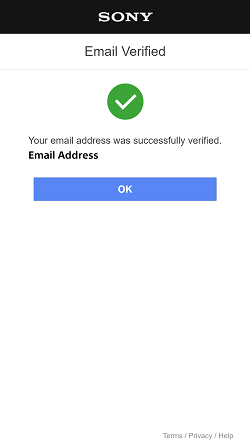The image showcases a mobile interface confirming the successful verification of an email address by Sony. At the top of the screen, the Sony logo is prominently displayed against a black bar with white text. Below the logo, a reassuring green check mark accompanies a message that reads, "Email Verified," followed by a confirmation statement: "Your email address was successfully verified." At the bottom of the screen, a blue "OK" button awaits the user's acknowledgment. The background is sleek and white, providing a clean and uncluttered look. Additionally, a footer at the bottom of the page contains links labeled "Terms," "Privacy," and "Help," offering users further assistance and information. This image illustrates a typical step in Sony's user verification process, ensuring that email addresses are authenticated, thereby preventing the creation of spam, bot, or troll accounts.